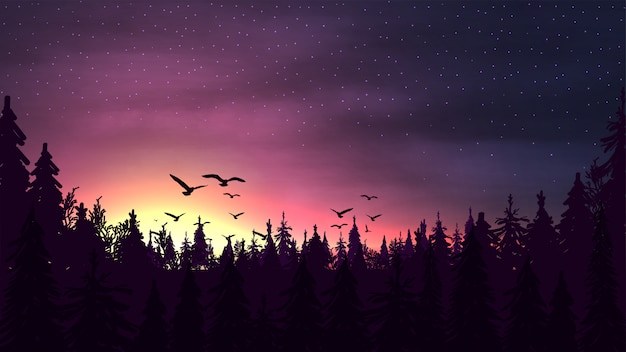A digitally created, rectangular image showcases a serene sunset over a pine forest. The bottom of the picture features the black silhouettes of evergreen trees, their tips forming a varied but mostly flat horizon. Moving upwards through the image, one encounters a group of approximately ten birds, arranged in small clusters, flying in triangular formations across a richly gradient sky.

The sky is the dominant feature, taking up the entire top half of the image and transitioning through a vivid spectrum of colors. Starting at the very top, the color scheme begins with a deep, nearly black purple, peppered with faint star-like dots and faint outlines of clouds. Lower down, this dark purple softens into lighter purples intermingled with pink hues. Just beneath the birds, the sky transitions to a warm yellow, indicative of the setting sun which has just dipped below the tree line.

Overall, the image captures a tranquil, almost mystical moment in nature with the stark contrast of dark tree silhouettes and the vibrant, fading light of the sunset.